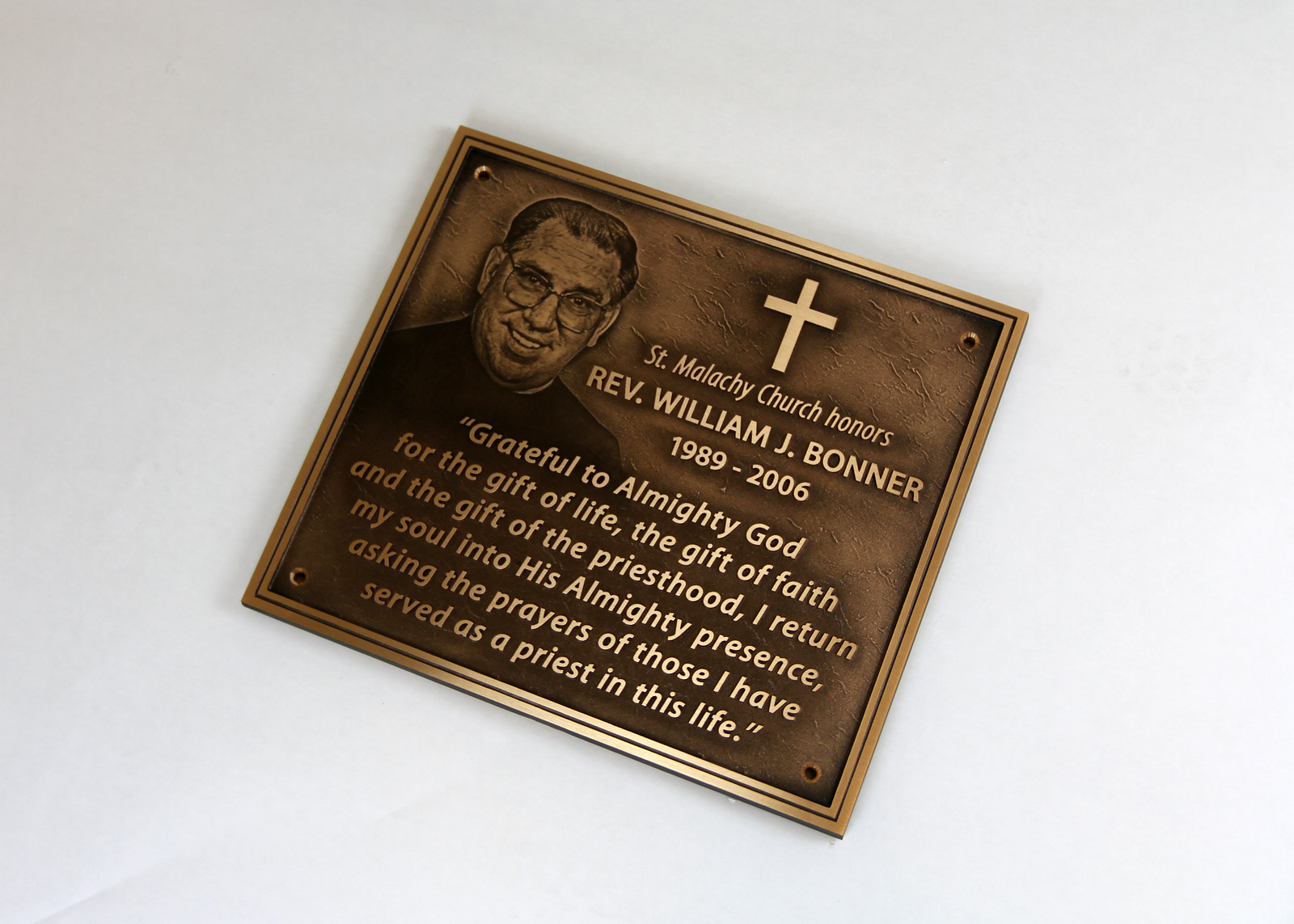The image depicts a bronze-colored square plaque with black framing, displaying a detailed black and white photograph of Reverend William J. Bonner, who is wearing glasses and a black shirt. At the top of the plaque is a cross, followed by the inscription: "St. Malachy Church honors Reverend William J. Bonner, 1989 to 2006." Beneath this, a heartfelt memorial reads: "Grateful to Almighty God for the gift of life, the gift of faith, and the gift of the priesthood. I return my soul to His almighty presence, asking the prayers of those I have served as a priest in this life." The plaque features four holes, one in each corner, indicating it is designed to be mounted, possibly on a coffin, mausoleum drawer, bench, or other memorial sites. This reverent tribute honors the former priest of St. Malachy Church, acknowledging his years of dedicated service and his passing.